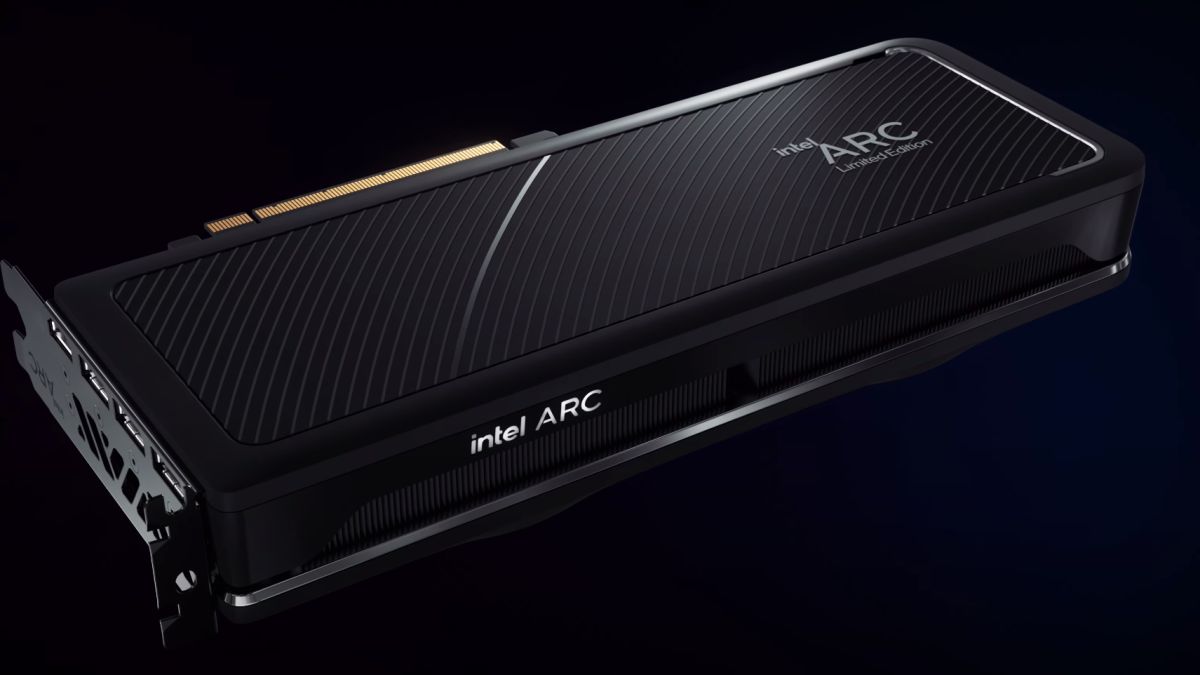The image showcases a sleek, modern piece of technology from Intel's ARC series. The device, predominantly black with "Intel ARC" emblazoned on the top, is designed with curved, diagonal lines that add to its sophisticated appearance. The device's dimensions and exact purpose are unclear from the image, but it could be a battery pack or a compact keyboard. Measuring details or scale is challenging due to the lack of reference objects. On the side of the device, "Intel ARC" is printed, and a series of ports are visible, potentially indicating connectivity options, possibly labeled with small symbols. Behind the main component, there appears to be a copper-colored connector, suggesting that the device may interface with other equipment, such as a computer or machinery. The entire setup is displayed against a black background, enhancing its contemporary design and rounded edges, emphasizing its high-tech, non-boxy construction.